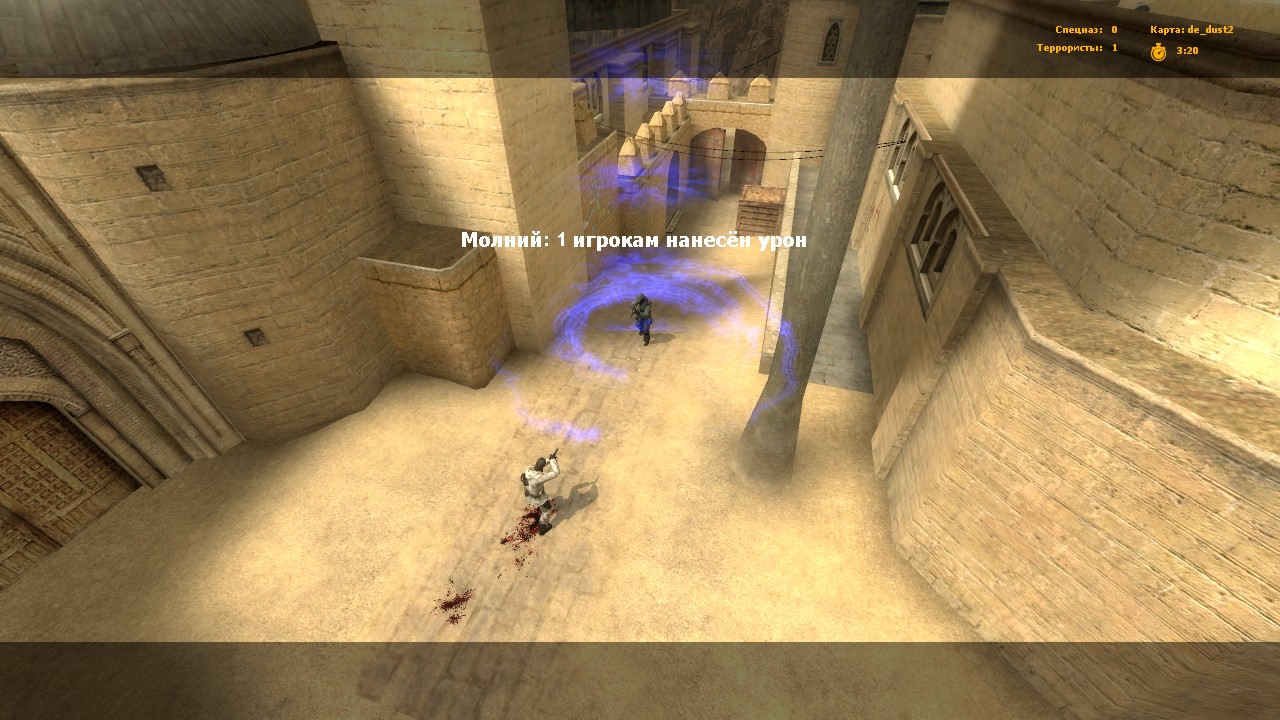The image is a detailed, horizontally oriented screenshot from a third-person shooter game, likely displayed on a wide TV. The scene depicted is inside a castle-like structure with tall stone walls, beige-yellowish in color, and a stone floor. A translucent brown strip frames the top and bottom of the image, with yellow text in possibly Russian or Ukrainian at the top right corner. 

Centrally, two figures are engaged in a confrontation. One figure, dressed in a white suit and wearing a brown helmet or mask, is situated at the middle left portion of the image. Blood is visibly splattered underneath this person, suggesting a recent injury or battle. This character is pointing a gun at another figure who stands directly at the center. Surrounding the central figure are blue, swirly mist or waves, giving an impression of some kind of energy weapon or special effect in use.

The structure features several carved areas, arched doorways, and columns, adding to the medieval castle ambiance. The evenly hued stone bricks and intricate detailing further emphasize the setting's ancient architectural style.